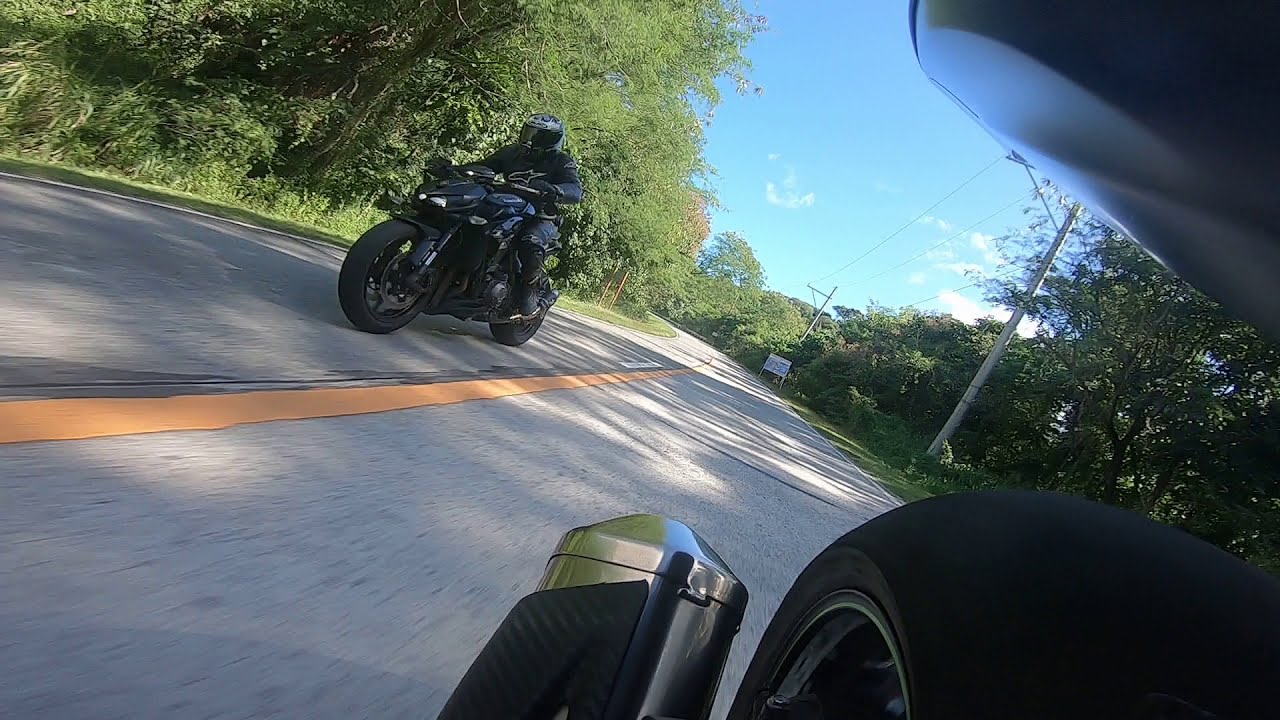The photograph captures two motorcycles on a well-lit, two-lane highway with a solid yellow line dividing the lanes. The scene is set on a partly cloudy day, with the clear blue sky peeking through. On the left side of the road, a motorcyclist dressed in an all-black outfit, including a helmet with a face shield, rides a black motorcycle. This rider's face is obscured by the helmet. The road is flanked by lush green trees and bushes on both sides, adding a natural backdrop to the scene.

The photograph appears to be taken from a camera attached to the rear of another motorcycle. This motorcycle's thick black rear tire is visible in the bottom right corner, along with parts of the top seat and the chrome silver exhaust pipe. You can also see some black hard plastic parts in the upper right corner of the image. Light poles are present along the roadside, likely to illuminate the highway at night. In the background, a sign stands amidst the trees, though its text is indistinguishable. Overall, the image portrays an open road adventure with two motorcyclists against the serene backdrop of nature.